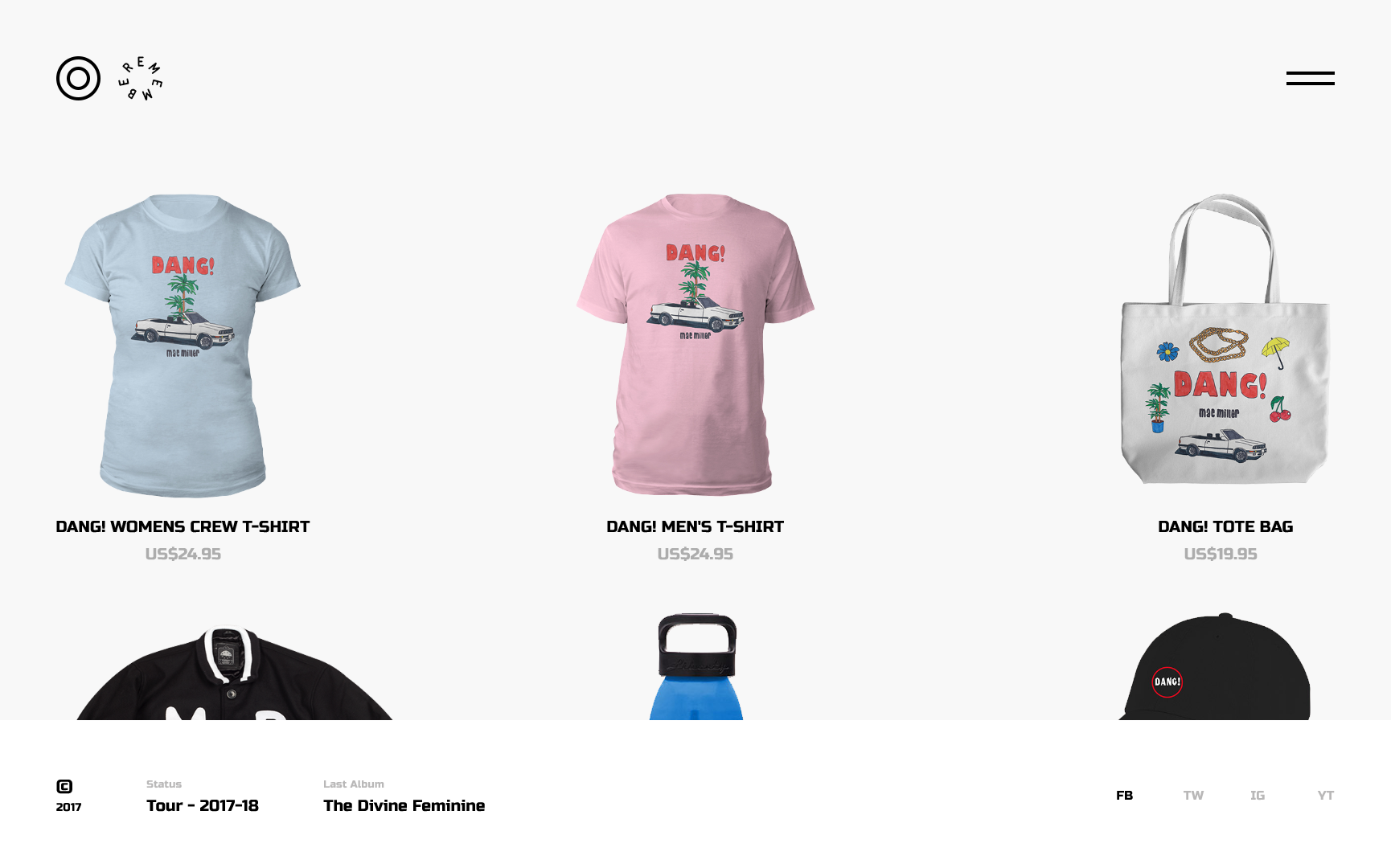The image features a light blue background. In the upper left corner, there is a circular emblem comprised of two concentric black circles with blue filling the space in between. Encircling the emblem are letters that seem to form the word "Member." To the right of this emblem, two black lines are visible.

Prominently displayed within the image are various items of clothing and merchandise. A blue t-shirt labeled "Dang Women's Crew T-Shirt" is priced at $24.95. Below it, a pink shirt labeled "Dang Men's T-Shirt" is also priced at $24.95. Additionally, a "Dang Tote Bag" is listed for $19.95.

On the right side of the image, there is a partially visible black jacket. Below this jacket, a small black handle attached to a blue object can be seen. Towards the bottom of the image, a black cap is present.

In the lower section of the image, there's a small black box displaying the text "C 2017/2018," accompanied by the phrase "The Divine Feminine." To the right of this box, the initials "FB" are visible, followed by three small buttons.